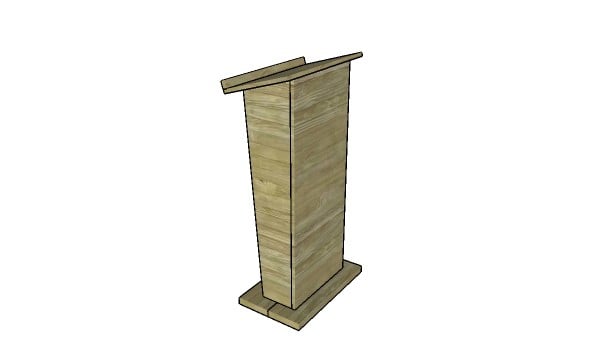This image features a computer-generated graphical artwork of a light brown wooden lectern positioned centrally against a stark white background. The lectern displays detailed wood grains and is framed by black outlines along its corners, base, and top. It stands on a base made up of two boards, with a vertical rectangular shaft that slightly widens towards the top. The top of the lectern includes a horizontally slanted board that tilts downward, with a thin bar running horizontally along its bottom edge, likely intended to secure pens or papers.